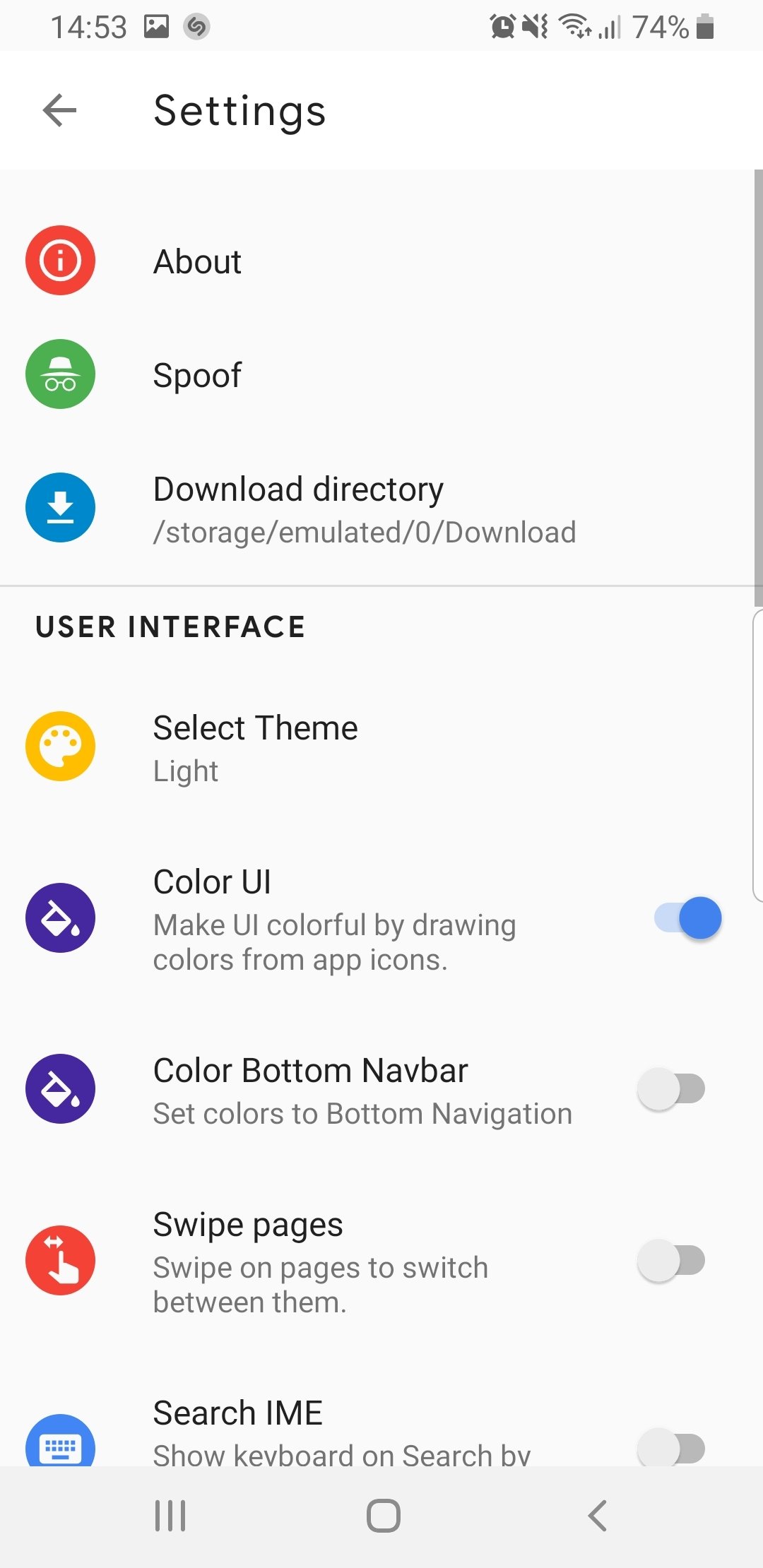The image depicts a screenshot from a cell phone, set against a solid white background. In the upper left corner, gray text displays the time "14:53." Next to this, the icon for the gallery photos app is visible. In the upper right corner, icons for an alarm clock, sound off, Wi-Fi signal, and a battery at 74% are displayed. Below these icons, the word "Settings" is written in black text.

Further down, there is a red circle accompanied by the label "About." Following this is the option labeled "Spoof" and beneath it, the "Download Directory."

A light gray horizontal line runs across the screen, under which the bold text "User Interface" is shown. Below this, the options "Select Theme" set to "Light" and "Color UI" are presented. The "Color UI" description reads, "Make UI colorful by drawing colors from app icons." At the very bottom, a toggle switch with a blue circle indicates that the toggle is turned on.